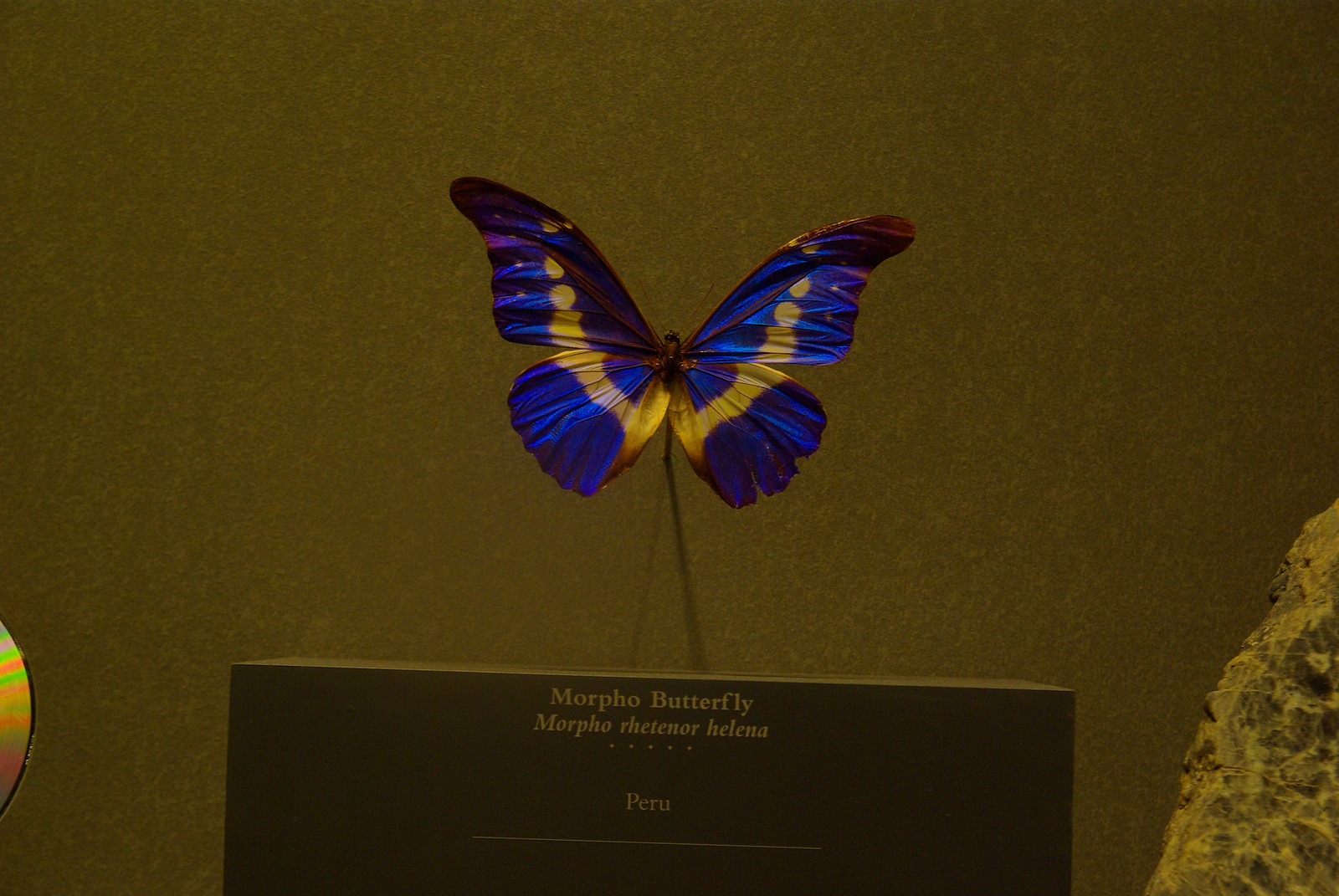In this image, we see a preserved Morpho butterfly displayed at the center against a bronze or brownish background. The butterfly features a striking bright blue body and wings adorned with yellow stripes running down each wing, and reddish-brown tips. The background also includes natural elements such as a rock on the bottom right and a reflective object, possibly a CD, on the bottom left. Below the butterfly, there is a dark-colored plaque with gold text that reads "Morpho butterfly," followed by its scientific name "Morpho retinor helena," and the mention of "Peru," indicating its native habitat. The light in the image appears to come from the top left, casting shadows behind the butterfly.